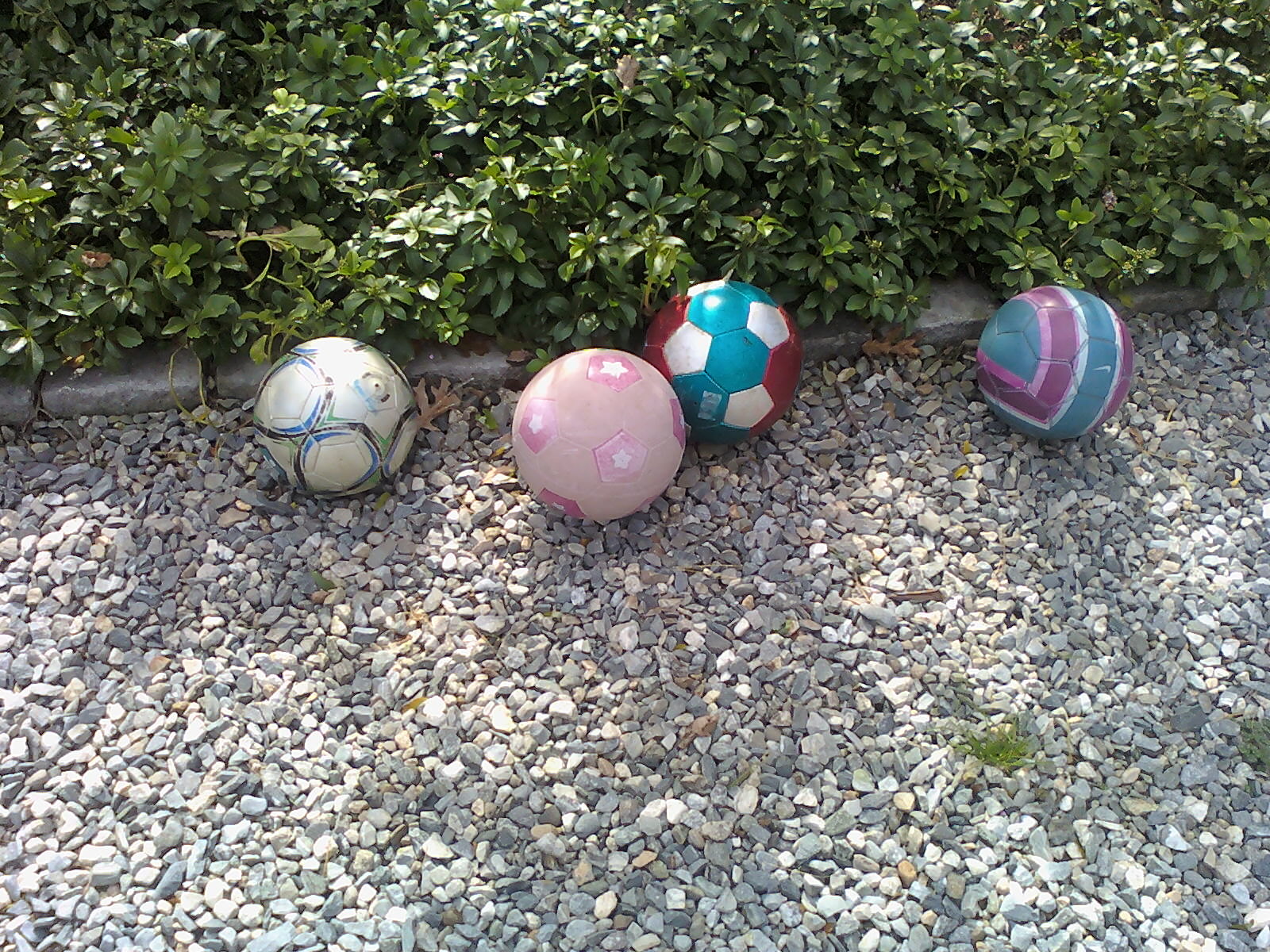This outdoor color photograph captures four soccer balls resting on a gray and white gravel path. The balls are placed almost in a row in the middle of the frame, against a background of gray stone curb bricks. Behind the curb, lush green foliage is visible, with the sunlight illuminating parts of the leaves. 

The first ball on the left is predominantly white, adorned with blue and green circular swirls. The second ball is light pink with darker pink hexagons that feature white stars in their centers. The third ball is a vibrant mix of turquoise, dark red, and white hexagons, giving it a multicolored appearance. The fourth ball, which appears slightly conical due to its stripes, features muted medium blue, deep pink, lighter pink, and white stripes, creating a unique pattern. Small bits of green grass peek through the gravel in the foreground, adding a touch of nature to the scene. The background also includes shadows from trees, adding depth to the image.